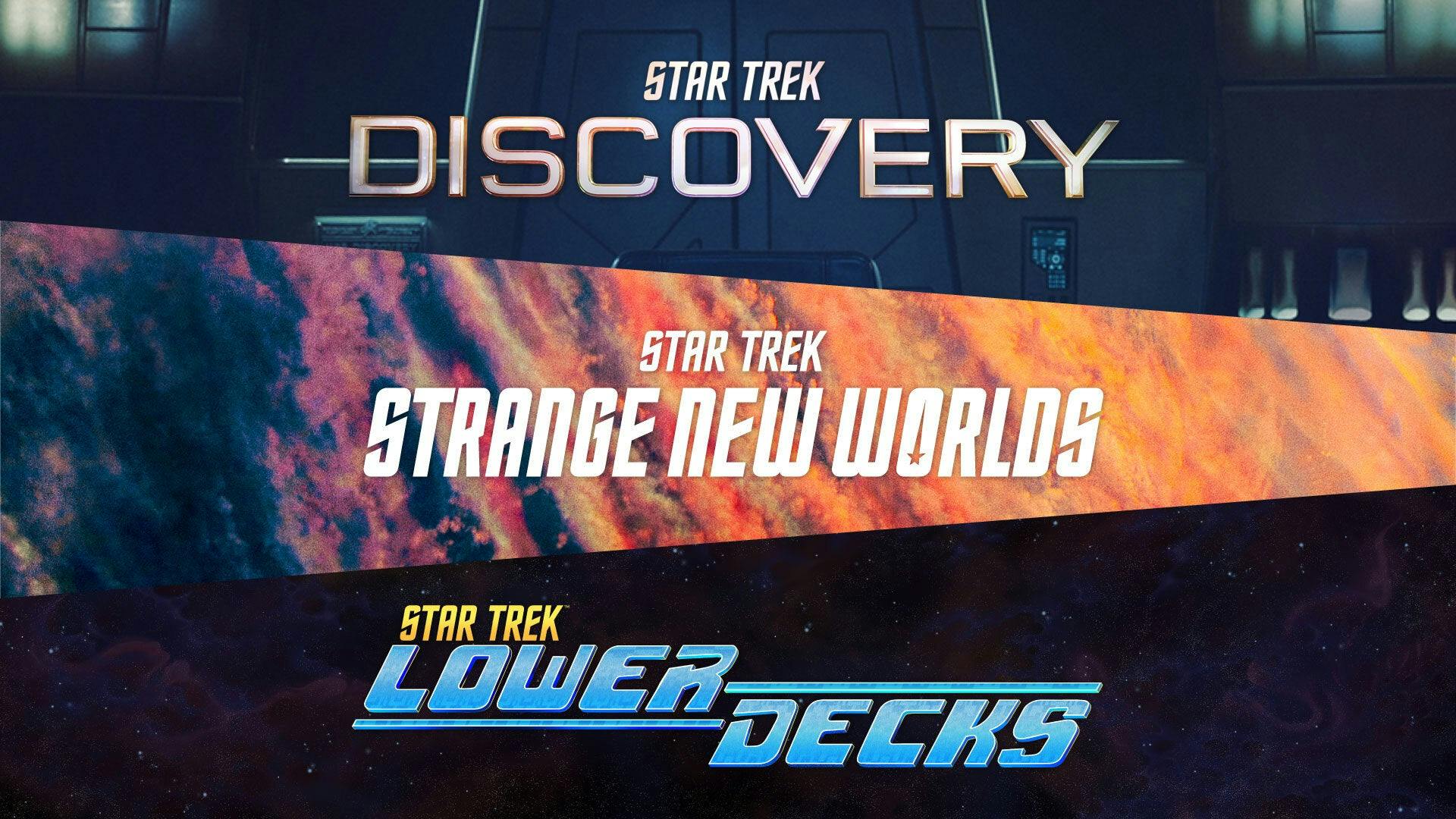In the image, there are three vertically-aligned posters, each representing a modern Star Trek series available on Paramount+. The first poster at the top features "Star Trek Discovery" written in white letters. The background shows a sci-fi door, likely representing a building's entrance, with bluish-grey walls. The middle poster displays "Star Trek Strange New Worlds," also in white lettering. Its background is vibrant, resembling colorful clouds with hues of blue, pink, orange, and yellow, along with a hint of an orange planet. The bottom poster showcases "Star Trek Lower Decks," where "Star Trek" is in yellow and "Lower Decks" in blue. The background depicts a vast expanse of outer space, filled with stars and purple-blue space clouds against a black sky. These posters collectively highlight the three contemporary Star Trek series, emphasizing their titles and thematic backgrounds.